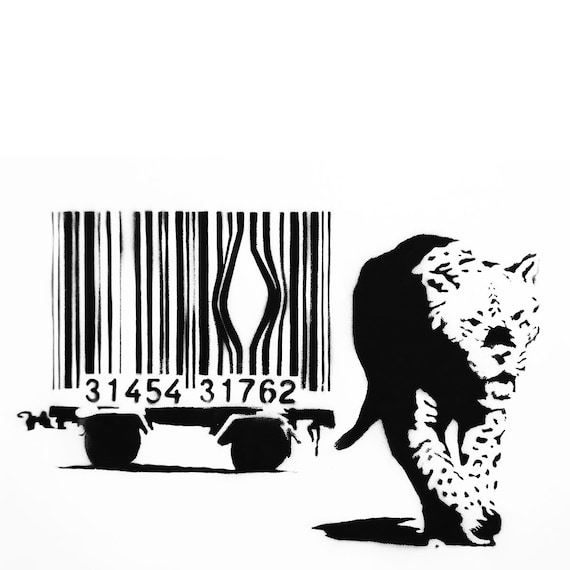The computer-generated black and white image depicts a dramatic scene with a silhouetted tiger on the right-hand side. The tiger is partially obscured in shadow, yet its face, front paws, and spots on the head are clearly visible. It appears to be striding forward, having just escaped from a barred cage on the left-hand side, resembling a circus train caboose. The cage's bars resemble a barcode, marked with the numbers 31454-31763, and have been pried open where the tiger has made its exit. The overall composition juxtaposes the vivid detail of the tiger against the stark, symbolic structure of the cage, evoking a sense of freedom and rebellion.